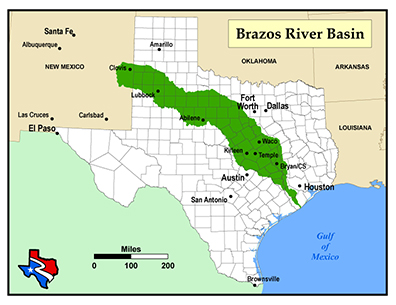This image features a detailed map of Texas, prominently displayed in white with discernible county lines marked in gray. Major cities such as Amarillo, Lubbock, Abilene, Fort Worth, Dallas, Waco, Temple, Bryan, Houston, Killeen, Austin, San Antonio, and Brownsville are identified by black dots and labels. Stretching diagonally across the state, from Clovis in the northwest to near the Houston area in the southeast, is a vivid green shaded region, indicating the Brazos River Basin, as stated in a bone white rectangular box in the upper right corner. The map also includes parts of neighboring states—New Mexico, Oklahoma, Arkansas, and Louisiana—depicted in a tan background. Additional features include the Gulf of Mexico in blue in the lower right, a scale indicating distances from 0 to 200 miles on the left, and an inset in the lower left showcasing a stylized depiction of Texas with a red, white, and blue design.